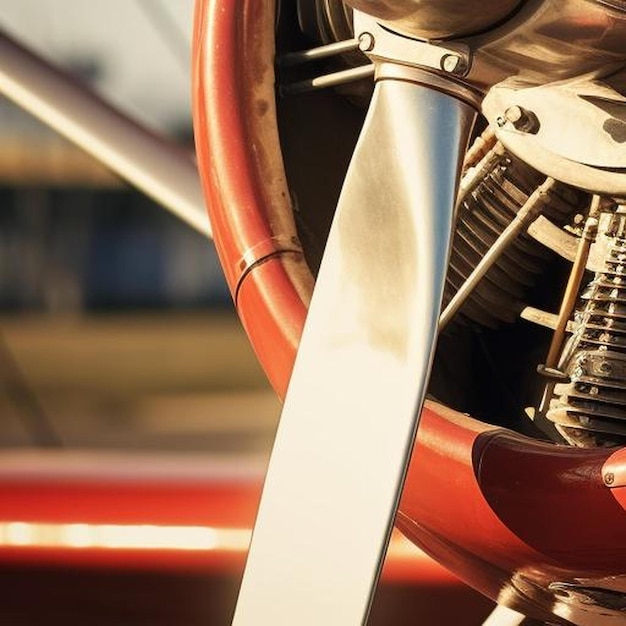This is a detailed, close-up photograph of a personal, single-motor biplane's propeller. The propeller is silver, and you can see approximately three-quarters of it, with the top, rounded portion left to the viewer's imagination. The aircraft itself is red or possibly a rust-colored orange around the engine cowling, with a curved, circular housing featuring a smooth array of screw-like pegs extending outward from the center, likely securing components together. The image also reveals part of the radial engine behind the propeller, characterized by pistons arranged axis-symmetrically around the main propeller shaft. The background, although blurred, appears to suggest an outdoor location near a hangar, illuminated by late morning or early afternoon light. Additional details include a visible part of the wing on the right side of the aircraft, along with a gray spar and wire supports indicative of a biplane's structure.